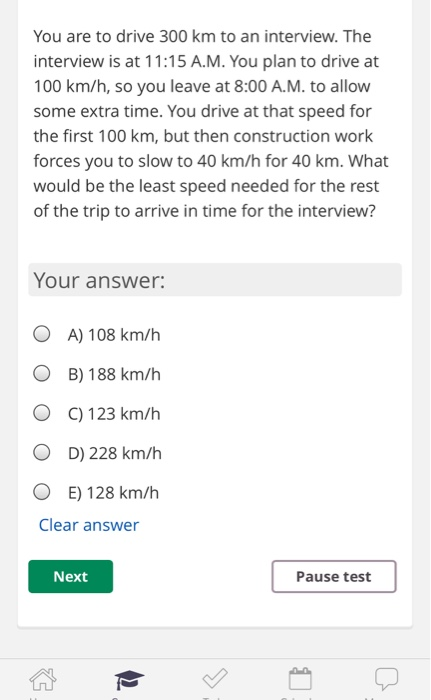This image is a narrow, vertically oriented screenshot of a question from an online quiz, likely taken from a smartphone. The background is pale gray, and within it is a white, rectangular area containing the quiz content.

At the top of the white rectangle, there is a question written in dark gray text: "You are to drive 300 km to an interview. The interview is at 11:15 a.m. You plan to drive at 100 km/h, so you leave at 8:00 a.m. to allow some extra time. You drive at that speed for the first 100 km, but then construction work forces you to slow to 40 km/h for 40 km. What would be the least speed needed for the rest of the trip to arrive in time for the interview?"

Directly beneath this question is a light gray banner topped with the text "Your answer:" in dark gray. Below this banner are five multiple-choice options, each with a tick box:
- (A) 108 km/h
- (B) 188 km/h
- (C) 123 km/h
- (D) 228 km/h
- (E) 128 km/h

Towards the bottom of the image, there is blue text labeled "Clear answer," likely a link to clear any selected options. On the left side, there is a green button with white text reading "Next." Adjacent to it on the right is a white button with a grayish-purple border and dark grayish-purple text that reads "Pause."

At the very bottom of the screenshot, there are partially visible icons, each indicating different functionalities: a home icon, a graduation cap, a checkmark, a calendar, and a chat icon.